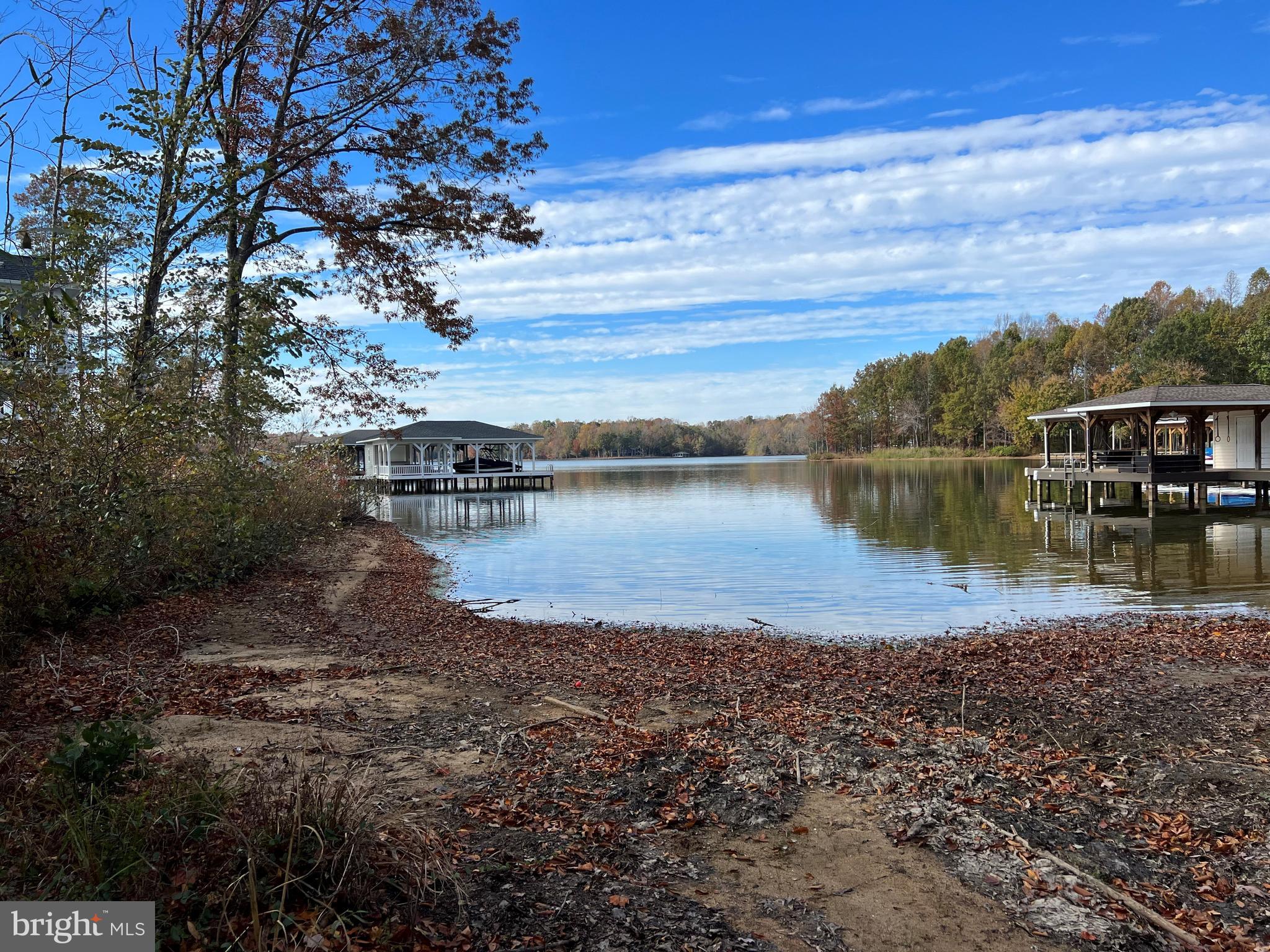The photograph captures a tranquil, outdoor scene during the daytime, featuring a large, reflective lake. The upper portion of the image showcases a blue sky adorned with long strands of white clouds. Far off into the background, the horizon is lined with green trees. Dominating the mid-ground of the photo, the vast lake mirrors the surrounding trees, adding a serene, glassy appearance to the water.

On the left side of the image, a white boathouse stands atop the lake, supported by numerous white columns and featuring a grayish, slanted roof. The foundation is made up of wooden bases that extend into the water to provide stability. There appears to be a boat docked within this structure.

Conversely, on the right side, another structure with a grayish roof is visible. This building is mostly brown and similarly elevated over the water on stilts, resembling the left side's boathouse but with subtle differences in design.

Closer to the foreground, the edge of the lake transitions into shallow water, littered with dead yellow and orange leaves, brown dirt, and occasional rocks, giving a rustic touch to the setting. On the left side, two large trees are prominent, adding to the natural ambiance. At the bottom left corner of the photograph, there is a gray rectangle with white print that says "Bright MLS."

In summary, the image beautifully captures the peaceful coexistence of natural elements and man-made structures, featuring a pristine lake flanked by unique boathouses, trees, and a clear blue sky.